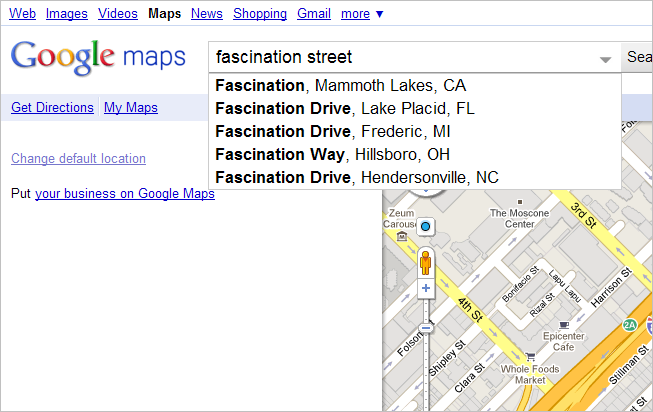This image from Google Maps displays a detailed "Fascination Sheet," highlighting recently searched destinations. The top five locations include Monmouth Lakes, California; Lake Placid, Florida; Frederick, Michigan; Hillsborough, Ohio; and Hendersonville, North Carolina. The interface offers functionalities such as obtaining directions, accessing personalized maps, and adjusting default location settings. There’s also a prominently featured invitation to add your business to Google Maps, emphasizing its value as a marketing strategy. A map of an unspecified area is also displayed within the interface.